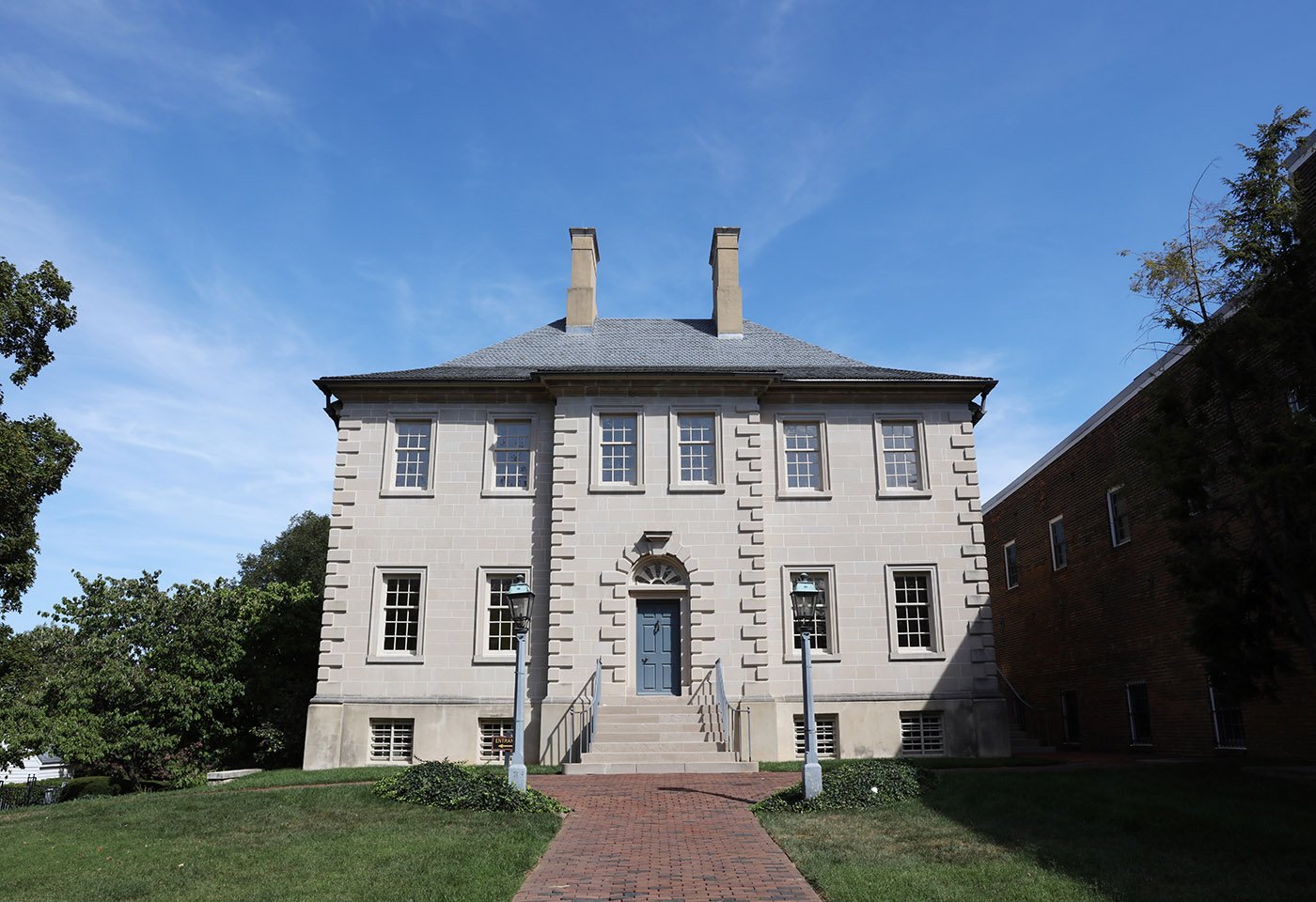The image is a digital daytime photograph of a residential two-story house made of light gray, large rectangular bricks. The house features an asymmetrical facade with six windows on the top floor and four windows on the first floor, all set into white frames. A red brick pathway with a slight upward slope runs from the bottom center of the image towards the house, flanked by a freshly mowed green lawn. Near the end of the pathway, on either side, there are light blue-painted street lamps set on silver poles. The pathway leads to concrete steps with light blue-painted rails that match the house’s front door, which is light blue and set into a white door frame beneath a small archway. The house has a sloped roof in light bluish-gray, with two tan-colored chimneys on top. To the right of the house stands a two-story red brick building with a flat roof. The background includes a blue sky with wispy white clouds and trees visible to the left of the house.